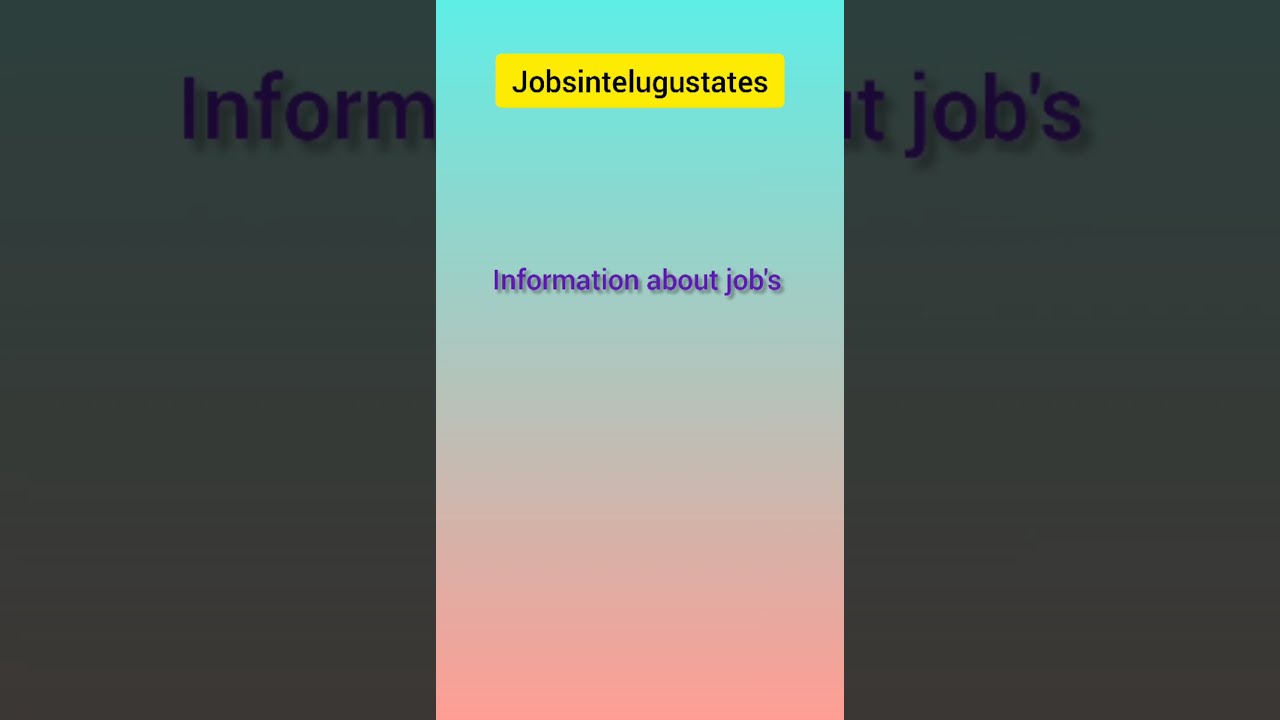The image is a simple graphic featuring a central, vertically-oriented rectangle with a gradient that transitions from turquoise at the top to peach at the bottom. This central section is framed by two semi-transparent, black layers on the sides, which magnify portions of the central text, converting the overall layout into a landscape format. 

At the top of the central rectangle, there is a yellow horizontal block with black text that reads "Jobs in Telugu States," spelled J-O-B-S-I-N-T-E-L-U-G-U-S-T-A-T-E-S. Slightly below this, the phrase "Information about Jobs" appears in purple text, with "Jobs" including an apostrophe 's' (Job's). In the background of the graphic, the same phrase, "Information about Jobs," is enlarged and darkened, creating a repeating and magnified effect on both the left and right sides of the image. The gradient effect in the background changes colors from a dark turquoise at the top to a pinkish-gray towards the bottom, contrasting subtly with the central gradient section.